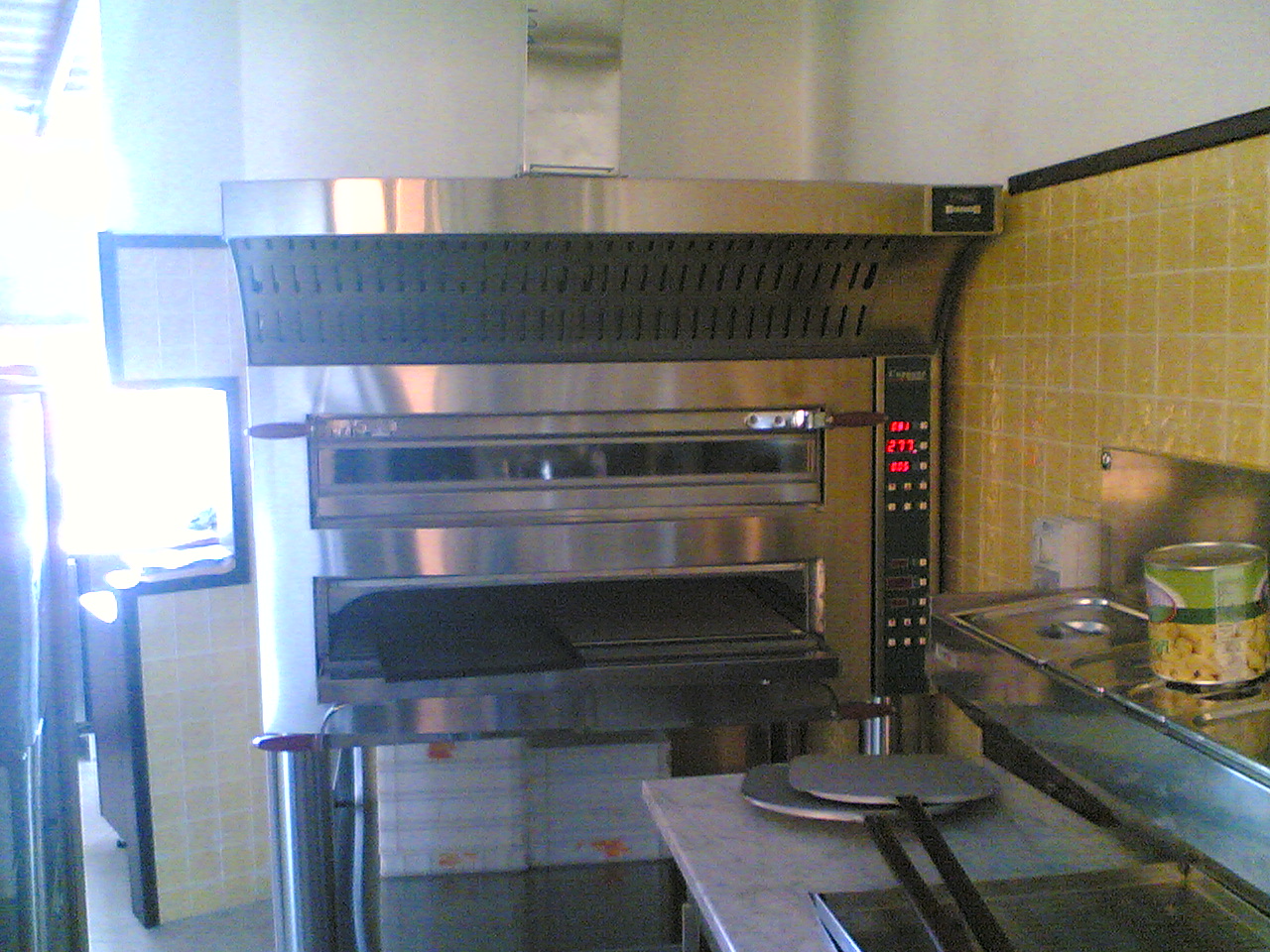This photograph captures a detailed view of a commercial kitchen, likely belonging to a pizza parlor or Italian restaurant. Central to the image is a large, stainless steel pizza oven with two slots – the top one closed and the bottom one open. The oven's control panel is on its right side, displaying red digital numbers: 001, 277, and 100. The surrounding walls are adorned with square yellow tiles that transition to white higher up. To the right of the oven, metallic counters and shelving dominate the scene, with a couple of pizza paddles, featuring black handles and silver blades, resting on the lower counter. An industrial-sized can with a green and yellow label sits atop the counter. Through a path leading out to the left, a window floods the space with natural light.